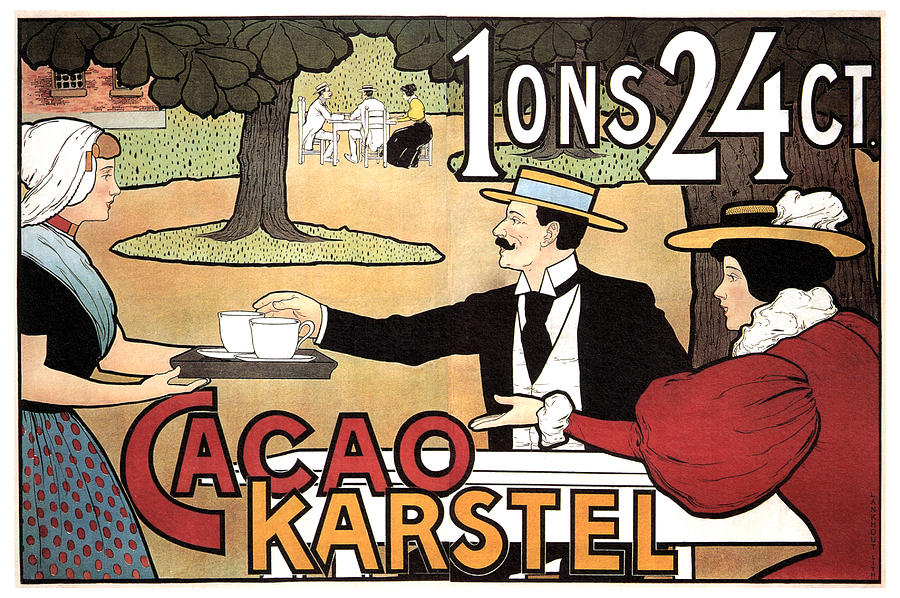A finely detailed, vintage-style advertisement for "Cacao Carstel" captures a lively park scene reminiscent of the Victorian era. At the heart of the image, a stylishly dressed man in a black suit, white vest, and black tie, topped with a distinctive stovepipe hat with a blue band, extends his right hand toward a white cup on a tray. His slender mustache curls upwards, adding a villainous flair. To his left, a woman in an elaborate red dress with puffed sleeves and white ruffles reaches out for the other cup on the tray. She sports a matching stovepipe hat adorned with a white ruffle accent and her dark hair contrasts with her fair skin. 

In the background, a server, wearing a green dress with red polka dots and a blue-green sash over a black top, holds the wooden tray with two large white coffee cups. Her head is wrapped in a white fabric headpiece, with strands of brown-blonde hair peeking out. Around them, the park setting unfolds with a large, brown tree to the right, its green-brown leaves providing a canopy. Behind the main figures, another table hosts two men in white suits and stovepipe hats, accompanied by a woman in a black dress bottom and yellow top.

The advertisement's ornate font "Cacao Carstel" arches at the top, with the letter "C" artfully swirling around the ensuing "A". Further textual details include "1 ONS" and a prominent "24CT" in the top right corner, indicating the product's premium quality. The scene is set against a backdrop of vibrant green foliage, a peach-colored ground, and a red brick building, completing the charming tableau.